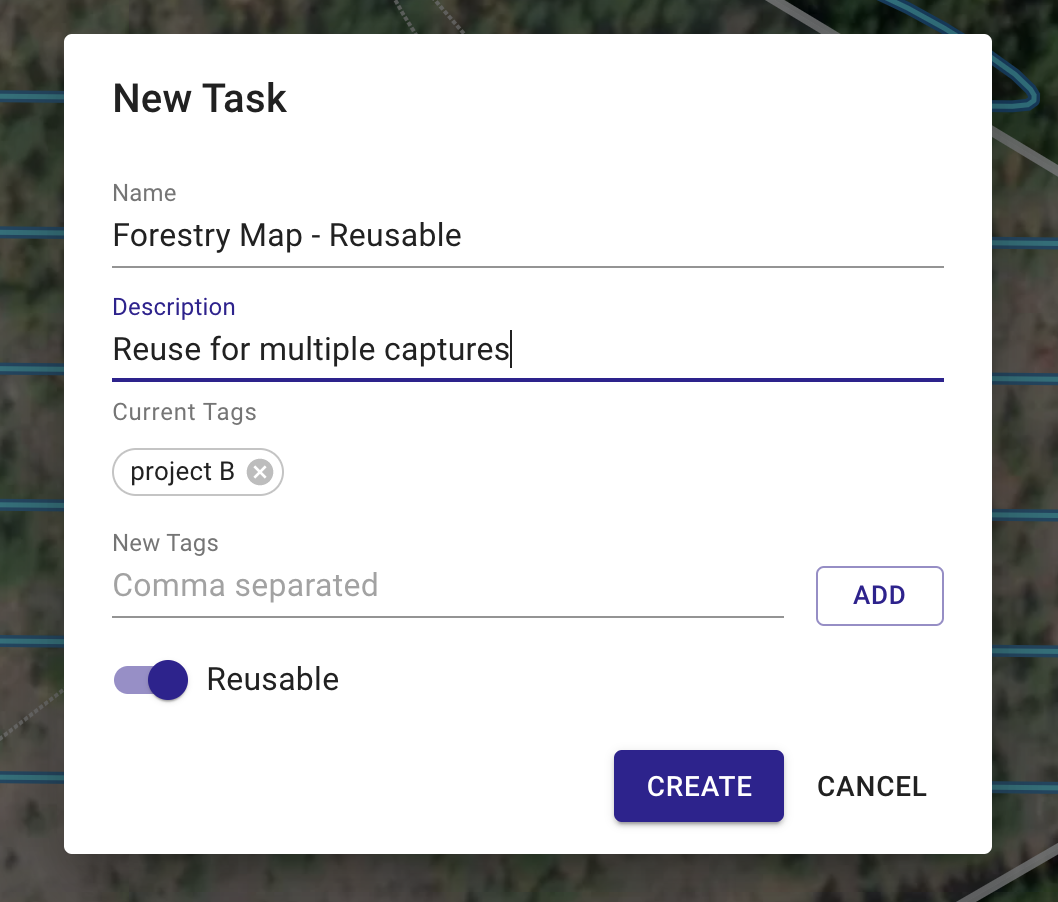The image depicts a user interface screen for creating a new task, set against a predominantly blackish-gray background accented with blue stripes. The central focus is a white square where the detailed interface elements are displayed. At the very top of this square, the words "New Task" are prominently written in black letters. There is a space for the task name, which in this example reads "Forestry Map - Reusable." Following this, a description field notes "Reuse for multiple captures." The section for current tags lists "Project Be," whereas the new tags field is empty and contains a placeholder in purplish-gray text that reads "comma separated."

Beneath the tags section, the word "Reusable" appears again in black letters, next to a slid purple toggle button indicating that the task is set to be reusable. On the right-hand side, there is a square button labeled "ADD." At the very bottom of the interface, there are two prominent options: a purple block displaying the word "Create" and a gray text option "Cancel." Additionally, the text "Reuse for multiple captures" is highlighted by an underlining purple line, emphasizing its clickable nature.